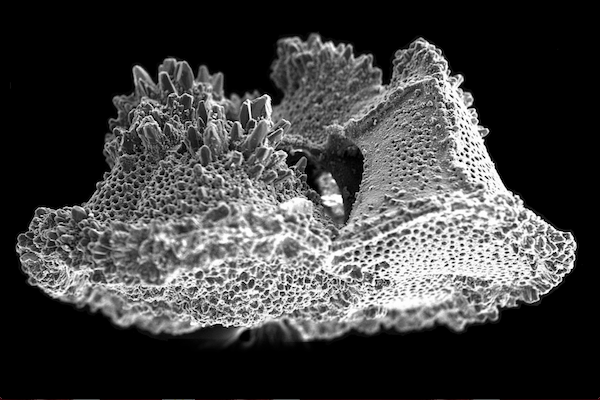This black and white image depicts an unidentifiable object under a microscope, featuring a complex structure reminiscent of coral or a natural crystal formation. The dominant black background contrasts sharply with the grayscale object, emphasizing its intricate details. The object itself rises towards the top, forming spiky, crystal-like protrusions reminiscent of jagged mountain peaks or coral formations. Scattered across its surface are numerous small, crater-like divots or pores, adding to its textured appearance. Central to the structure is a distinct, dark, hollowed-out ring that draws the eye, with the sharpest focus and highest definition in the image's center, leaving some peripheral areas intentionally blurred for depth. The detailed portrayal suggests a high-resolution microscopic examination, capturing the fine nuances of this enigmatic specimen.